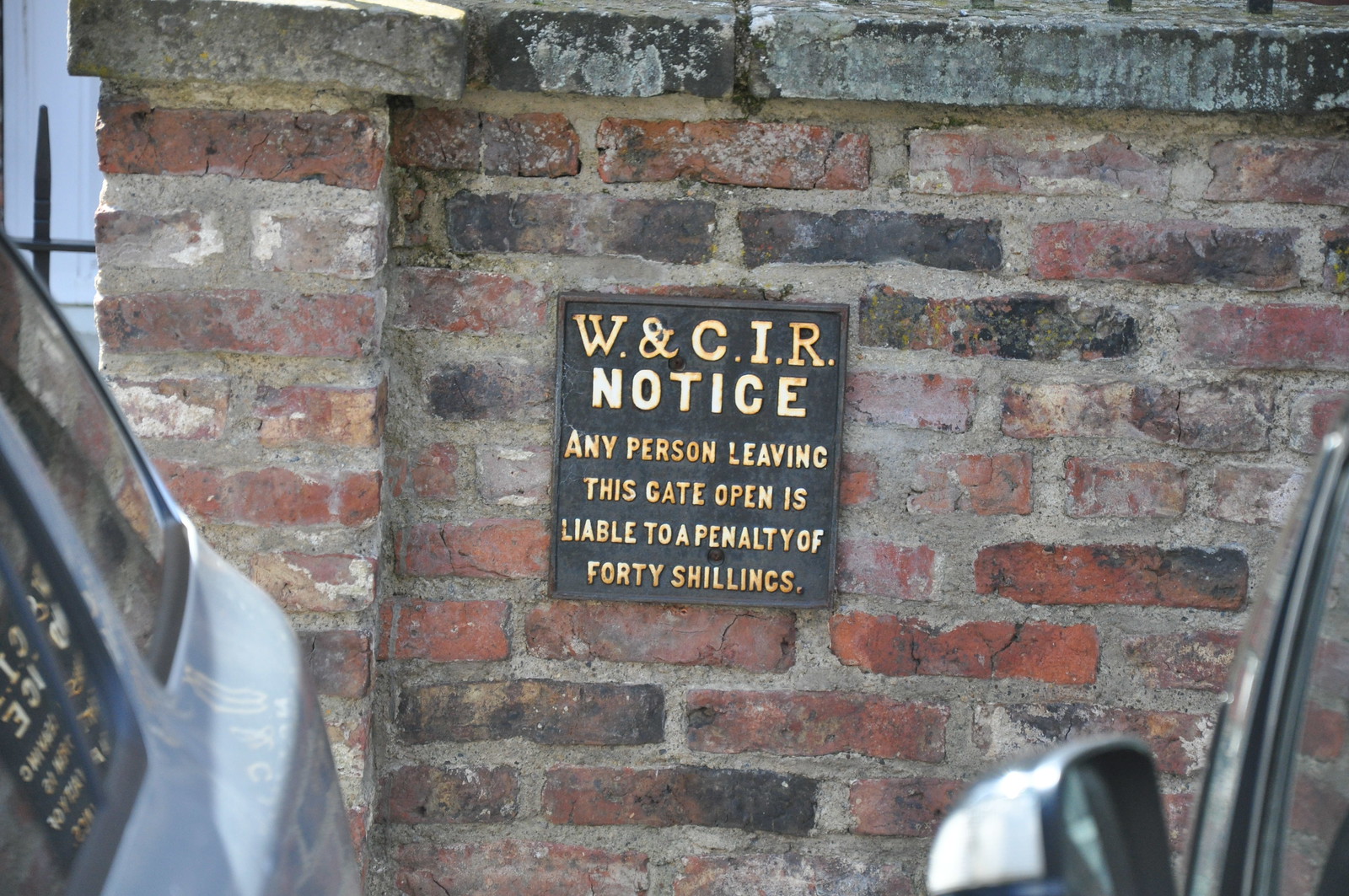The image is a horizontally aligned rectangular photo featuring an old, weathered red brick wall, interspersed with gray and black bricks. The focal point of the image is a dark brown metal sign affixed to the center of the brick wall. The sign, which bears gold lettering, reads: "W & C.I.R. NOTICE: Any person leaving this gate open is liable to a penalty of 40 shillings." Additionally, the image includes partial views of a vehicle; the lower right corner shows a side mirror and window, while the lower left corner reveals what appears to be part of a back window and the vehicle's white paneling. The photo appears to be taken outdoors during the daytime.